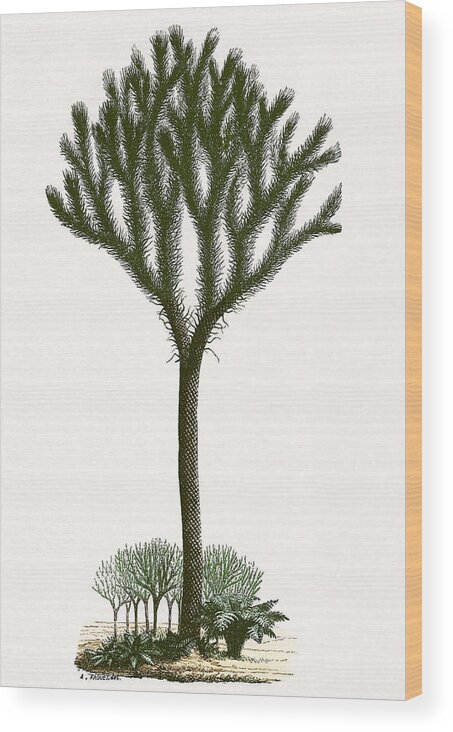This is an extremely detailed painting, resembling a piece of wall art, illustrating a solitary, tall Joshua tree against a solid white background. The tree features a long, intricately textured trunk akin to pine needles or a scaly, pinecone-like surface. Its branches at the top are tightly condensed, sprouting sharp, needle-like leaves. The painting also includes several more barren trees and bushes at the base of the Joshua tree. The trees in the background seem distant, enhancing the still-life composition. The artwork is created on a faux wood panel with a light gray-brown trim around the edges, contributing to its depth—about an inch thick—with a drop shadow cast down and to the right, suggesting it's mounted or displayed in a mock-up style. The canvas lacks any textual elements, focusing solely on the stark, almost pricking texture of the branches against a light yellow dirt ground.